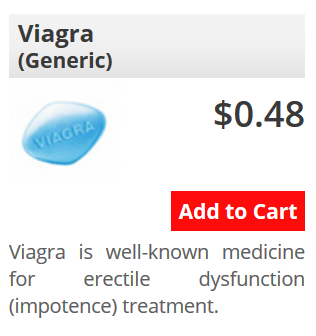This is a screenshot from an online medical site featuring a selection of drugs, including prescription medications available at discounted prices. The header prominently displays "Viagra," with "generic option" noted in brackets beneath it. Below the header, the brand name "Viagra" appears again, indicating the name-brand version of the drug. The image also shows a blue, diamond-shaped pill priced at 48 cents each.

The text next to the pill reads, "Viagra is a well-known medicine for erectile dysfunction (impotence) treatment." This panel appears to be part of a larger website, likely focused on selling generic drugs online, although it may offer a variety of medications.

The site’s language is in English and prices are listed in dollar signs, suggesting it could be oriented towards an American audience, although its specific origin is unclear. There are concerns about the legality of purchasing such medications without a prescription within the US, raising questions about regulatory compliance. Despite this, sites like these operate due to possible legal loopholes, providing Americans—and potentially individuals worldwide—access to these medications.